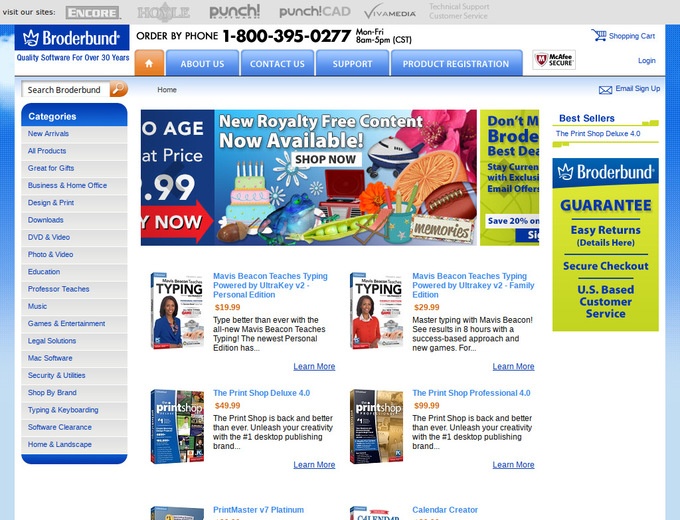This screenshot depicts a dated interface for the Broderbund website. 

**Top Section:**
- **Logo:** Located at the top left, the Broderbund logo features a crown above the text "Broderbund" on a small solid dark blue rectangle.
- **Tagline:** Beneath the logo, the tagline reads "Quality Software for Over 30 Years."
- **Navigation Bar:** A gray bar at the top includes various links: "Visit Our Sites," "Encore," "Hoyle," "Punch," "Punch CAD," "Viva Media," "Technical Support," and "Customer Service."

**Order Information:**
- **Order by Phone:** Below the navigation bar is a section that provides a phone number for orders, along with their hours of availability.

**Primary Navigation Tabs:**
- A horizontal selection bar contains several tabs:
  - **Home Icon (Orange):** Indicates the current page.
  - **About Us**
  - **Contact Us**
  - **Support**
  - **Product Registration**
  - **McAfee Secure Icon:** Ensures secure transactions.
- **Shopping Cart:** Icon located to the right.
- **Login:** Button below the shopping cart icon.

**Main Interface:**
- **Search Bar:** Positioned above a list of categories on the left.
- **Ad Banner:** Centralized in the main content area.
- **Product Listings:** Below the ad are various software products, focusing on titles like "Mavis Beacon" (two products) and "The Print Shop" (two products). Prices are displayed in orange, with descriptive text in black and blue.

**Right Sidebar:**
- **Guarantee Section:** Offers assurances such as "Broderbund Guarantee," "Easy Return," "Secure Checkout," and "US-Based Customer Service."

**Overall Aesthetic:**
- Dominant colors are white and blue, contributing to a very busy and cluttered visual presentation.

This detailed description provides a comprehensive understanding of the website's layout, content, and overall look.